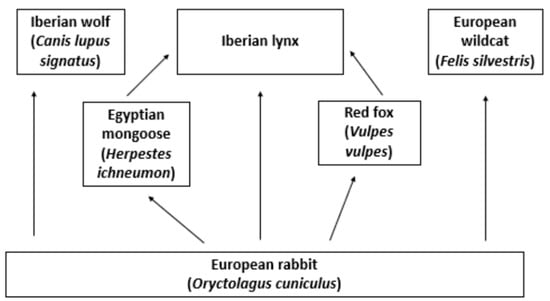The image depicts a black-and-white rectangular chart mapping out the relationships between various European animals through a series of interconnected arrows. At the bottom center, it starts with a large rectangle labeled "European Rabbit (Oryctolagus cuniculus)." Three arrows stem from this rabbit: two diagonal arrows lead to the middle of the chart, connecting to two rectangles; the left one for the "Egyptian Mongoose (Herpestes ichneumon)" and the right one for "Red Fox (Vulpes vulpes)." Both the mongoose and the fox have arrows that further lead diagonally upwards to a central rectangle at the top center, labeled "Iberian Lynx (Lynx pardinus)." Additionally, the European Rabbit has vertical arrows extending directly upwards to two top corners: the "Iberian Wolf (Canis lupus signatus)" on the top left and the "European Wildcat (Felis silvestris)" on the top right. All of these rectangles are interlinked with arrows, visually describing their connections within the ecosystem.